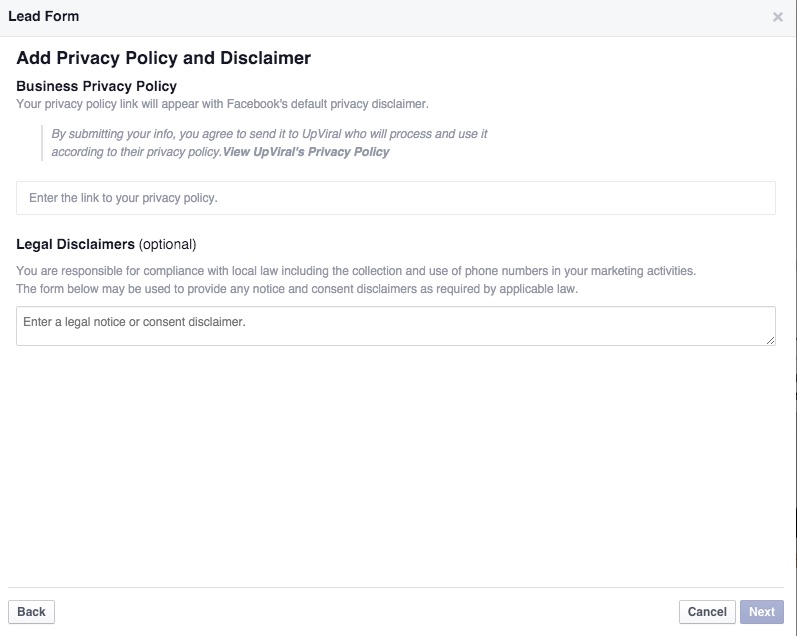In the upper left corner of the image, there is a lead form set against a light gray strip that extends horizontally across the entire width. On the right side of this strip is a prominent "X" button. Just below the strip, a section instructs users to "add privacy policy and disclaimer" with the text "Business Privacy Policy." It informs users that their privacy policy link will appear alongside Facebook's default privacy disclaimer and further explains, "By submitting your information, you agree to send it to UpViral, who will process and use it according to their privacy policy." There is also a prompt to view UpViral's privacy policy. The form includes a field labeled "Enter your link to privacy policy," followed by a section for a "Legal Disclaimer (optional)." A note below this field advises users of their responsibility for compliance with local laws, including the collection and use of phone numbers for marketing purposes. It mentions that the form below can be used to provide any necessary notices and consent disclaimers as required by applicable law and includes a data field labeled "Enter a legal notice or consent disclaimer."

At the bottom left corner of the image, there is a "Back" button, while on the bottom right corner, there are "Cancel" and "Next" buttons. The color scheme of the form is minimalist, employing black, gray, and white tones. The background is completely white, and the majority of the text is in gray, while headers and other significant information are displayed in black.